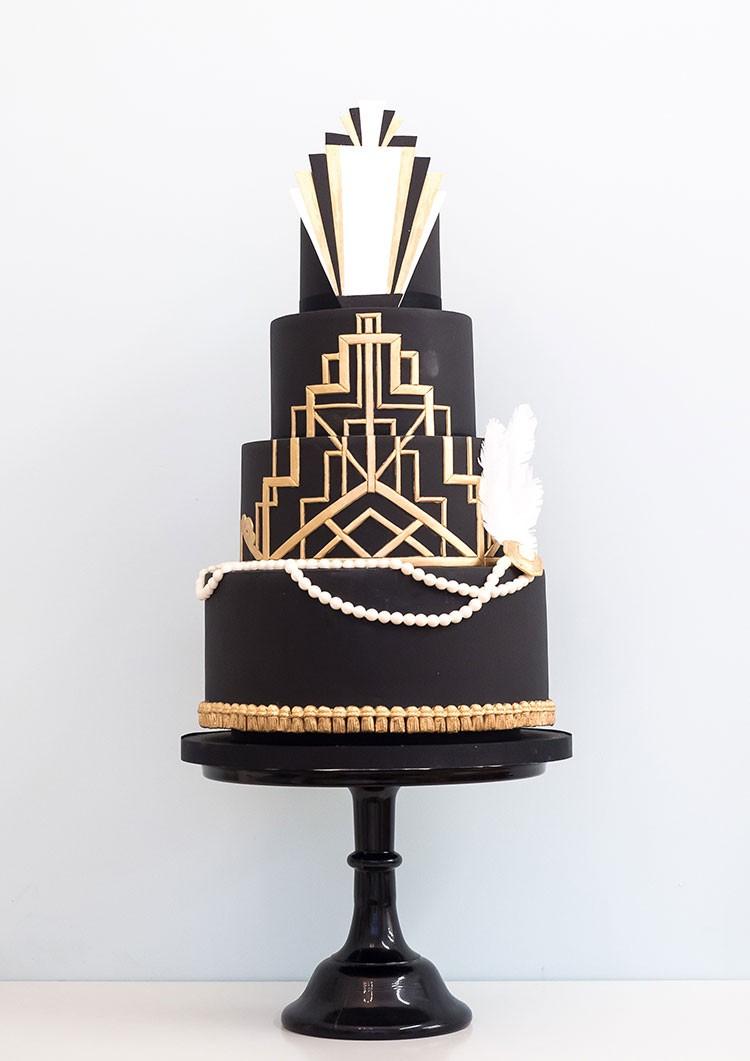This photograph features a highly detailed, modern-style, multi-tiered cake sitting on a black, circular stand that tapers off into a plunger-like shape. The cake primarily presents a matte black color palette adorned with intricate white and gold decorations. The bottom tier is embellished with gold tassels along its base and draped with white pearls adorning the top edge. Moving upwards, the second tier showcases a design reminiscent of an Art Deco building, with clean, geometric lines in gold. This design continues into the third tier, which further emphasizes the architectural motif with small, interlocking triangles forming a zigzag pattern. The fourth and final tier, which has a squared-off appearance with one side overlaid possibly symbolizing a present, is topped with a bow motif— the bow being predominantly chocolate brown bordered and beige, with a white center. The overall aesthetic is enhanced by additional details like white pearls flowing vertically down the second tier, resembling a strand of a pearl necklace, and a white feather protruding from the right side. The cake rests on a white countertop against a baby blue wall.